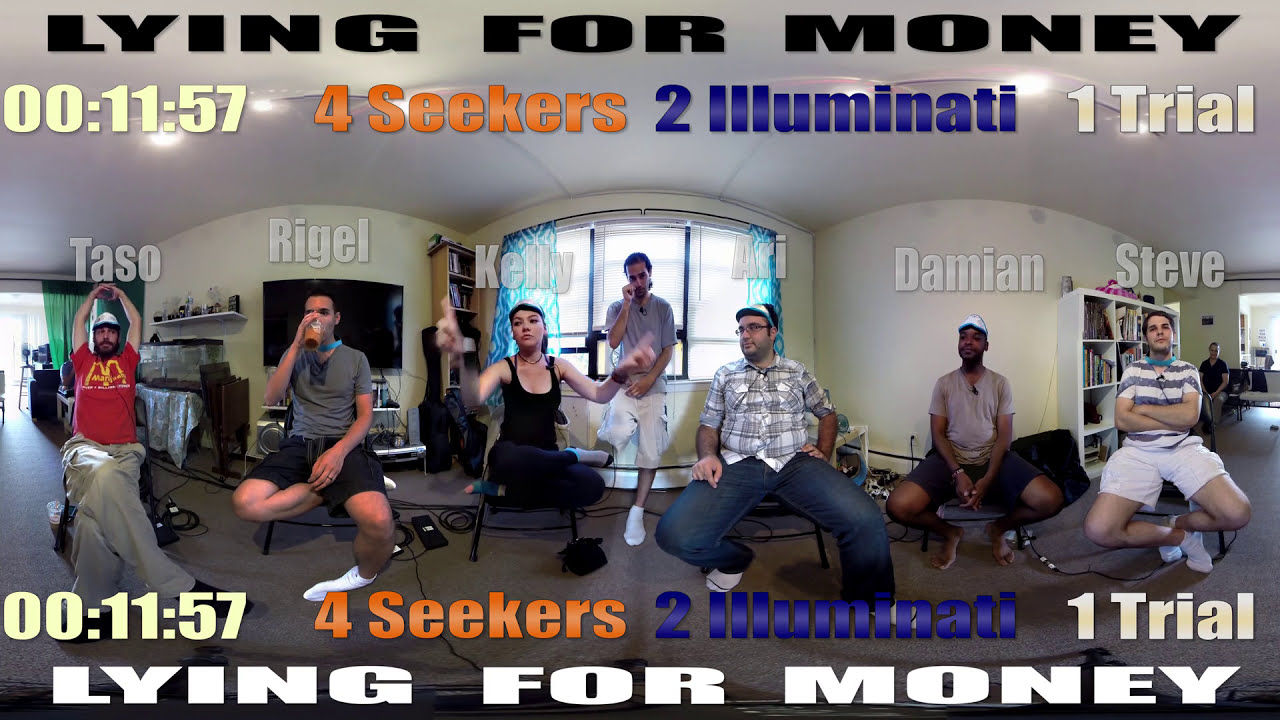In this vivid YouTube video thumbnail, the scene is set in a wide, panoramic view of a large room with curved walls and windows flanking either side. Seven young individuals, mostly men, are seated in black folding chairs, arranged in a semi-circle. Each participant has their name displayed above their heads from left to right: Tasso, Rigel, Kelly, Ari, Damien, and Steve. The central figure, who remains unnamed and stands in the background, appears to be observing rather than participating. The backdrop suggests a living room or game room setting.

Large text dominates the top and bottom of the thumbnail, proclaiming "Lying for Money." It includes a timestamp reading 11 minutes and 57 seconds. Highlighted phrases in bold colors announce the structure of the event: "Four Seekers" in red, "Two Illuminati" in blue, and "One Trial." The individuals are captured mid-action—gesturing, seated still, or possibly partaking in a game—implying a dynamic, interactive scenario. This elaborate setup hints at a live-streamed game show, involving elements of deceit and strategy.